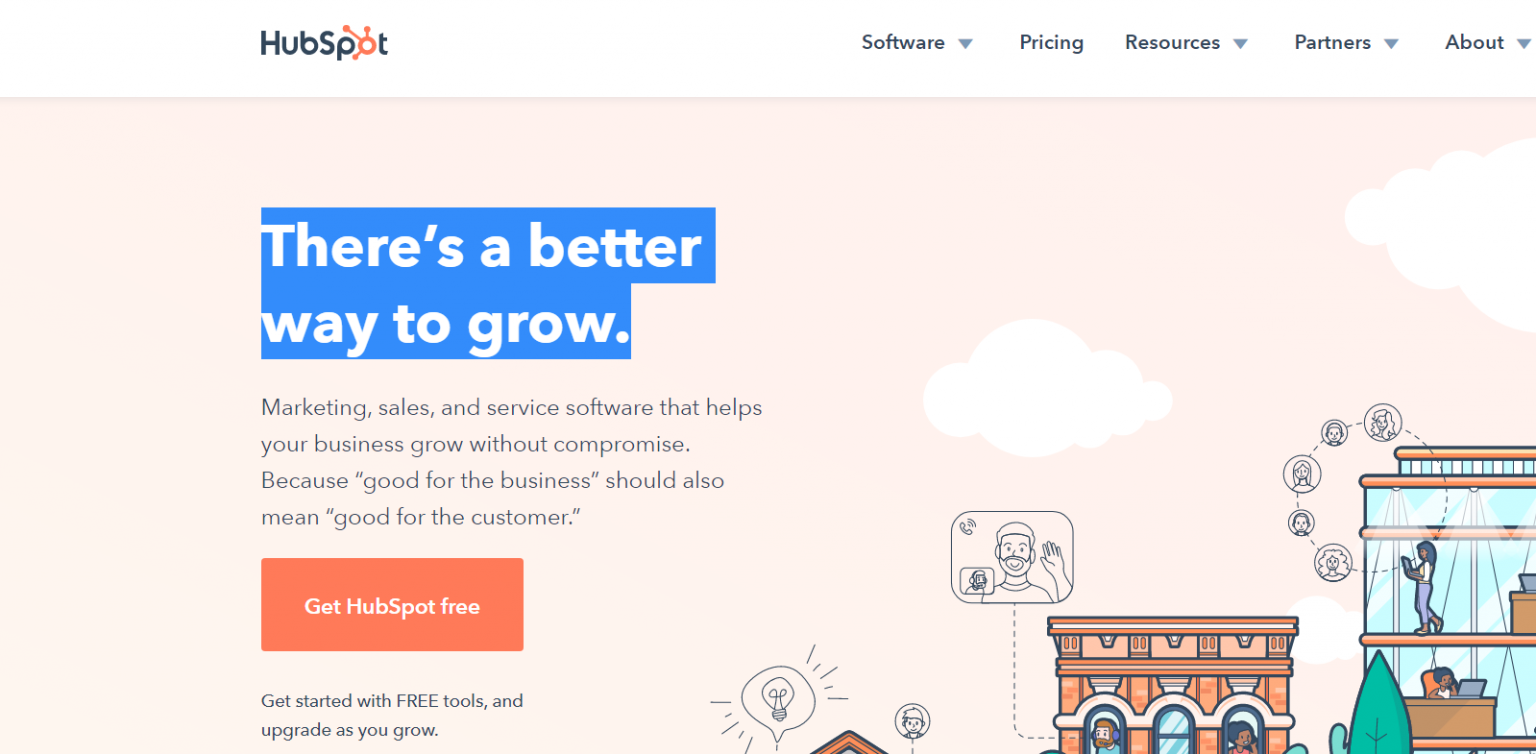In the top left corner of the image, the word "HubSpot" is prominently displayed, with the "H" and "S" capitalized in black letters. Notably, the "O" next to the "T" is orange with radiating lines, while the rest of the letters are black.

On the right-hand side, a series of clickable buttons are present. The options include "Software" in bold black text, followed by a gray downward-pointing triangle indicating a drop-down menu. This format is repeated for other buttons labeled "Pricing," "Resources," "Partners," and "About."

The center of the image features a peach-colored background adorned with white clouds and multiple buildings. To the far right, there is a brown building with blue window openings. Through these windows, one can see an individual working at a desk and another person walking away from the desk on the second floor. To the left, there is another building with a mix of brown, tan, and lighter brown colors. This building features a glass door flanked by two arches. A sign shows a person waving while seemingly holding a smartphone, possibly engaging in a FaceTime-like interaction. Lastly, a third building with only its orange roof visible has an idea light bulb icon popping up from it.

On the left side of the image, there is a dark blue Tetris-like shape featuring white text that reads, "There is a better way to grow." Below this, in black text, it states, "Marketing, sales, and service software that helps your business grow without compromise. (Good for business should also mean 'good for customers')." An orange clickable button, with white text saying "Get HubSpot Free," is positioned beneath this message. Under this button, in black text, it says, "Get started with free tools and upgrade as you grow."